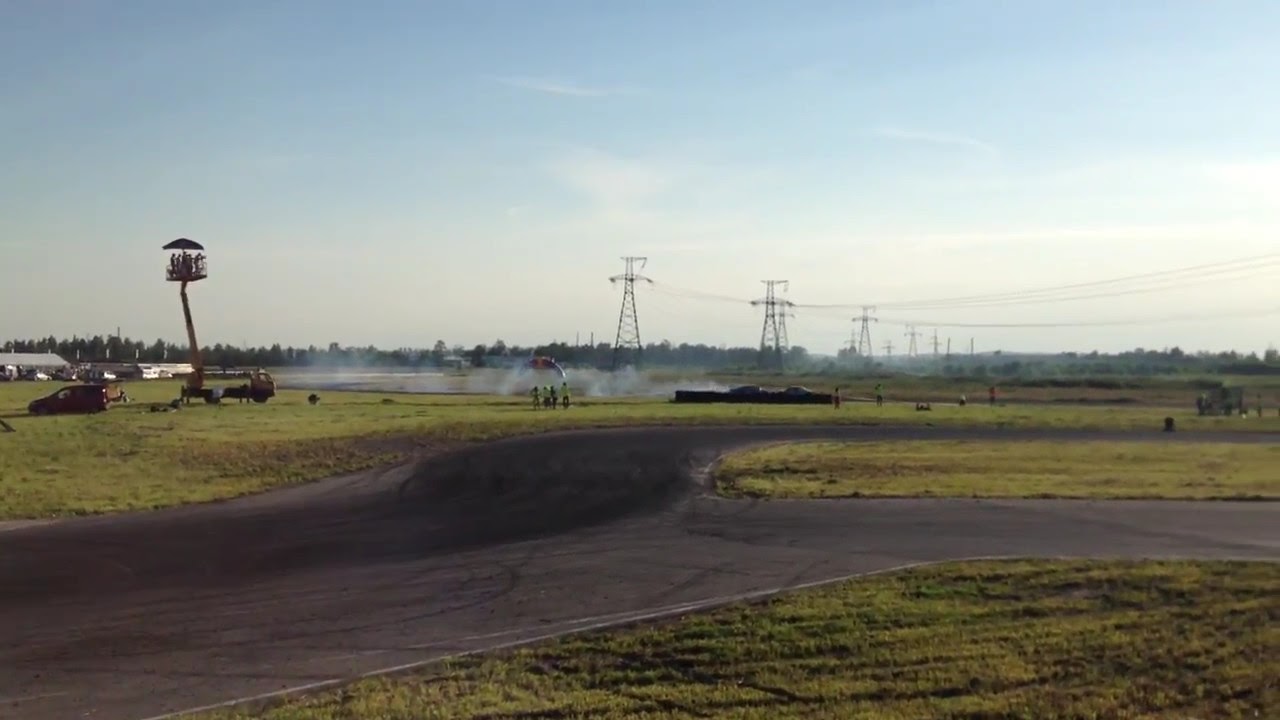The image captures an outdoor scene of a bustling racetrack. At the forefront, there's a black asphalt track branching off into two paths, creating a distinctive Y shape. The center of the Y and the immediate foreground are adorned with green grassy areas. To the left-hand side, a prominent yellow tower with an umbrella-like canopy stands tall, where people are gathered, presumably watching the races from an elevated vantage point. Tire marks are visible on the tarmac, indicating recent activity on the track, likely drifting, as suggested by the faint traces of cars and a cloud of tire smoke in the background. Beyond this, a row of white metal buildings is seen, and power lines along with towers rise above the landscape. Further into the horizon, a line of trees stretches across, and the sky above is a bright blue, interspersed with wispy clouds, and the overall scene is bathed in a bright, hazy light from the middle right of the image.